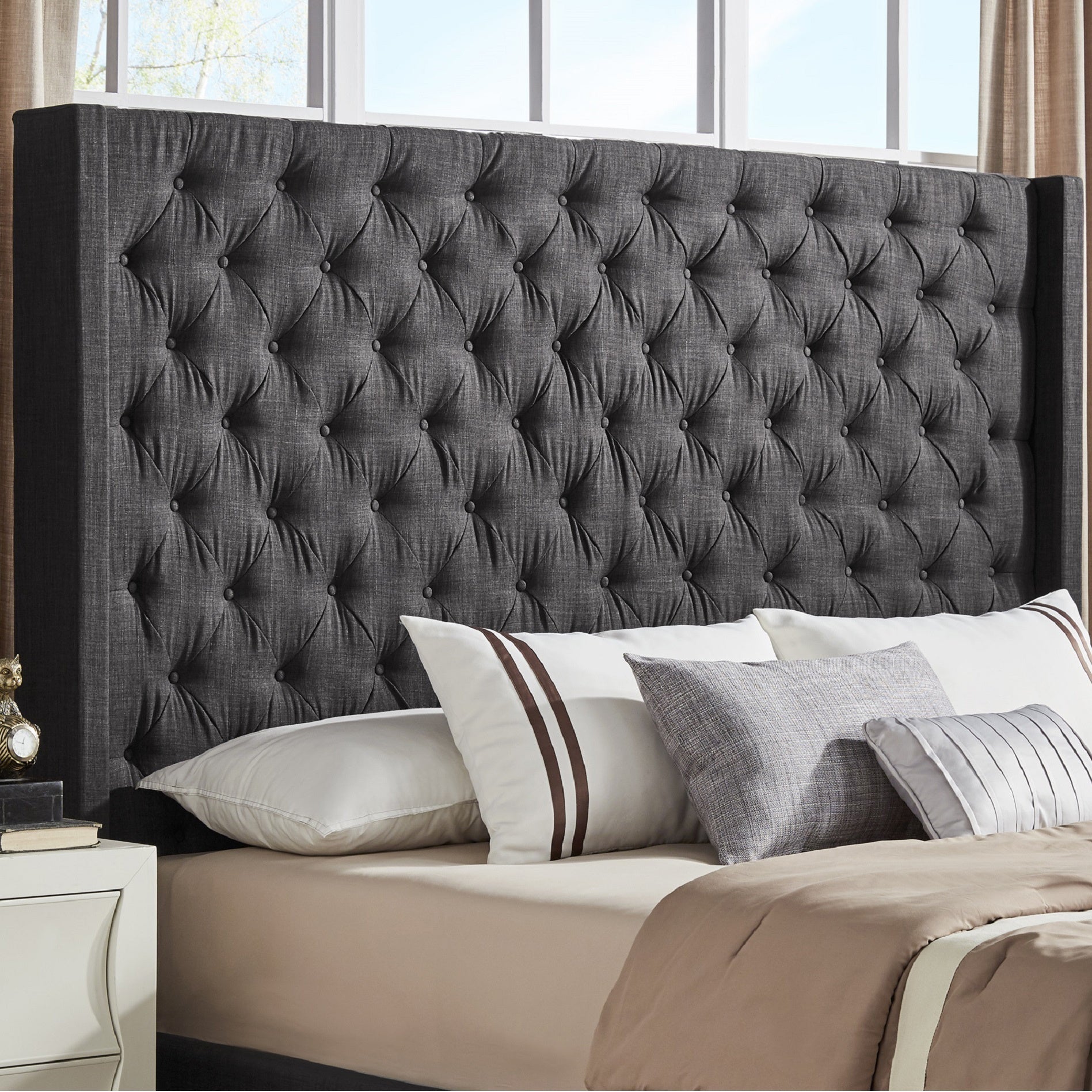The photo showcases a luxuriously appointed bedroom, likely from a high-end home or hotel. Dominating the scene is a towering, quilted headboard in dark gray, detailed with fabric buttons running across it, creating a sophisticated pattern. The headboard’s flat top and protruding side borders partially obscure a window draped in long, tan curtains with white window frames to the left.

The king-sized bed itself is dressed in opulent white and light brown sheets. Six pillows are meticulously arranged: two large white pillows lie flat, with two more white pillows, adorned with brown stripes at the ends, leaning against them. Two small gray throw pillows add a final decorative touch. Adjacent to the bed sits a white nightstand, playfully topped with a clock-faced cat, accentuating the room's blend of elegance and whimsy.